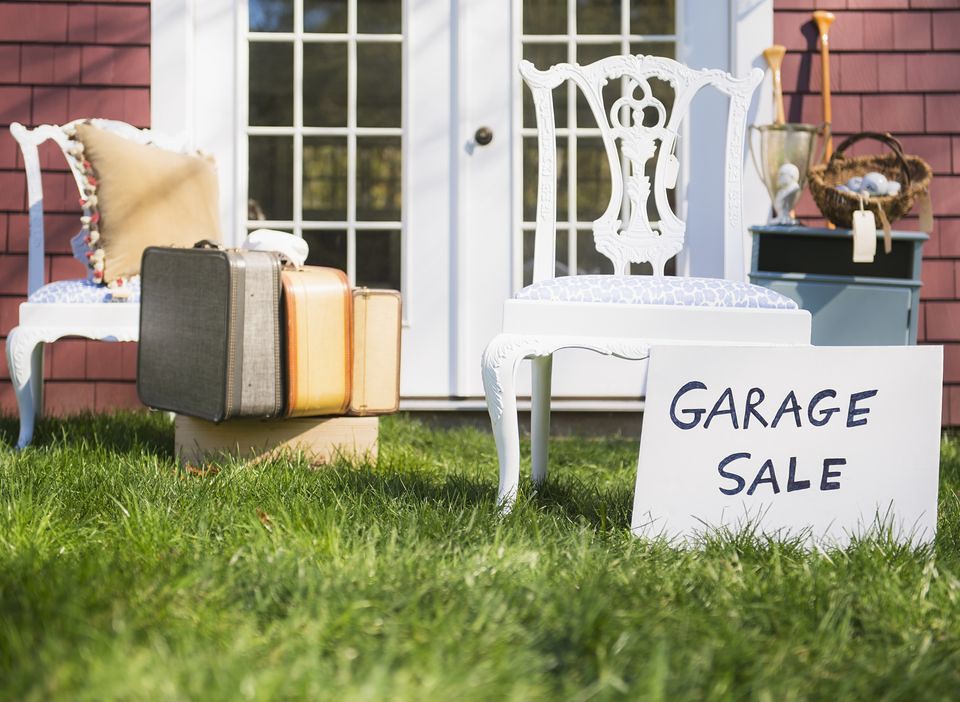The image showcases an outdoor garage sale set in a grassy yard on a bright day. The scene is filled with a variety of objects spread out across the yard. On the ground, lush green grass serves as the surface for displaying items. To the left, there is a tan cushioned chair adorned with tassels. In front of this chair, three vintage suitcases of varying sizes are stacked atop a cardboard box. Moving to the right of the suitcases, a white modern chair with a blue and white cushion leans against a sign that reads "garage sale". 

Behind this chair, a stand displays several items for sale, including a basket filled with plastic fruit and a silver trophy-like vase. In front of the vase is a small ceramic bust of a man. Leaning against the side of the house, which features red vinyl siding and two white double doors with clear window panes, are a couple of curtain rods and possibly some paddles for a boat. 

The overall color palette includes green, black, white, red, tan, gray, light blue, orange, brown, and reddish brown. The objects are dispersed throughout the yard without a central focus, enhancing the casual, eclectic feel typical of a garage sale. The setting is clearly outdoors, during the middle of the day, capturing the essence of a neighborhood event.